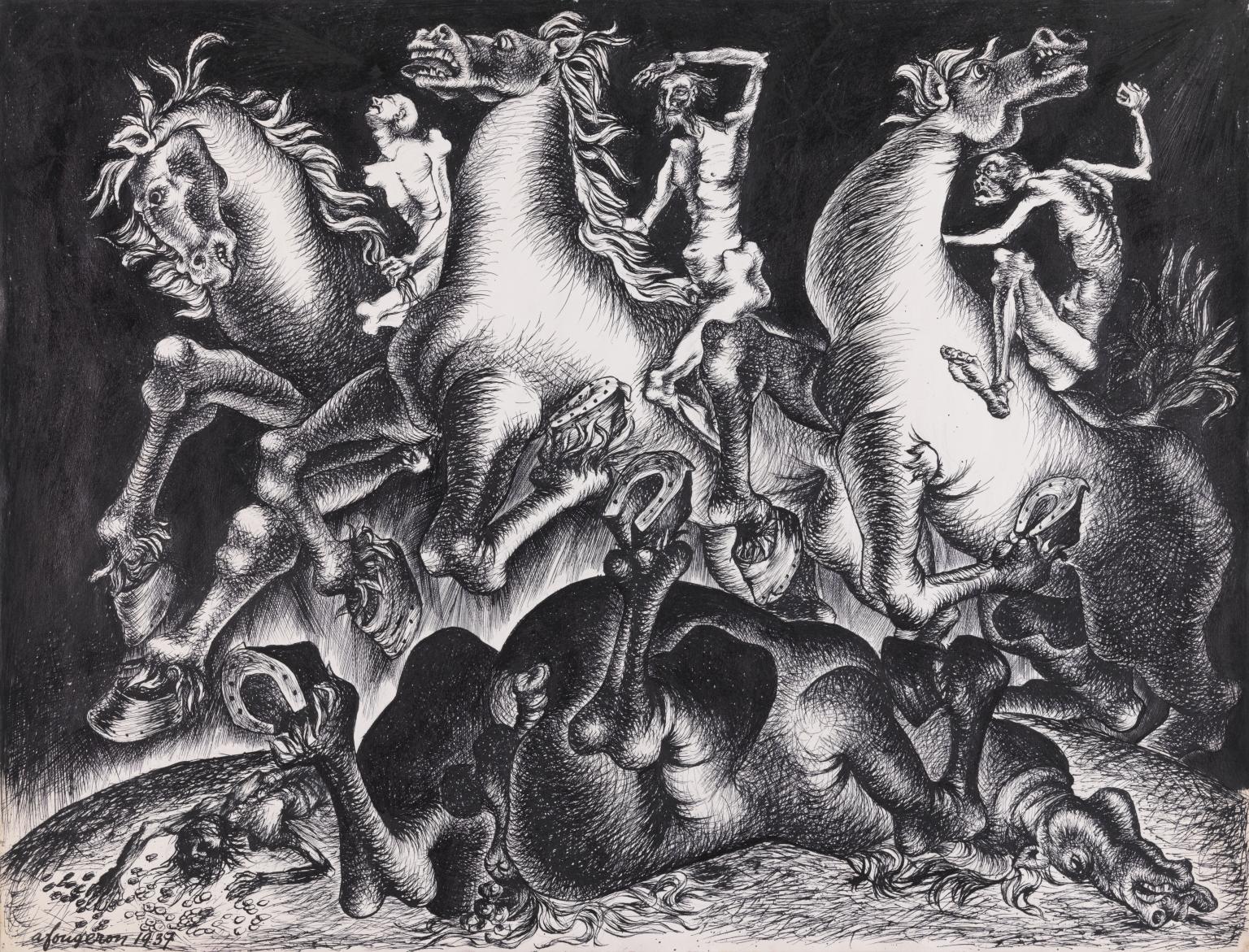The drawing depicts an eerie and haunting scene in black and white, set against a dark, chalky background reminiscent of a blackboard erased of white chalk markings. Foregrounded are three emaciated, almost zombie-like figures with their ribs prominently visible, riding horseback. The horses, depicted with a whitish hue, are reared up on their hind legs, appearing frightened. These skeletal riders, who seem devoid of clothing, exude an unsettling, demonic aura. Below them lies a black horse on its back, legs raised with visible horseshoes, its head slack and tongue protruding, suggesting death. Near the fallen horse is a figure on the ground, possibly dying. The image carries an ominous, medieval or biblical tone and is underscored by a barely legible cursive watermark that reads "a for Jerem" with the year "1937."